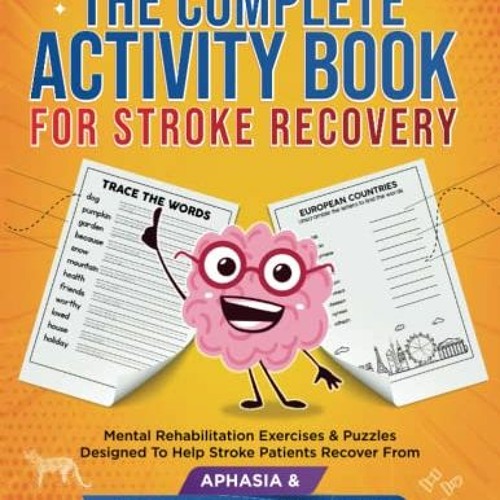The image is a bright and lively book cover designed for stroke recovery, featuring a yellow to orange gradient background with the center more yellow and the sides more orange. At the top, large blue text with a white outline reads "The Complete Activity Book," though the very top edge is cropped off. Below, in smaller red text with a gradient fill from bright to dark red, it reads "For Stroke Recovery." 

Centered on the cover is a whimsical, cartoonish brain character. The brain is pink and has a bubbly, almost bubblegum-like appearance. It sports red spectacles with big white circular eyes and a black and white smiling mouth. The character has simplistic stick arms and legs, one of which is pointing upwards.

Behind the brain character are two paper-like graphics. The worksheet on the left is titled "Trace the Words" and includes dashed lines for tracing words such as dog, pumpkin, garden, and others. The worksheet on the right reads "European Countries" and contains lines for filling in blanks with the names of countries.

At the bottom of the cover, small black text states, "Mental Rehabilitation Exercises and Puzzles Designed to Help Stroke Patients Recover From." This is followed by a skewed purple rectangle with white text reading "aphasia and," though part of the text appears cut off.